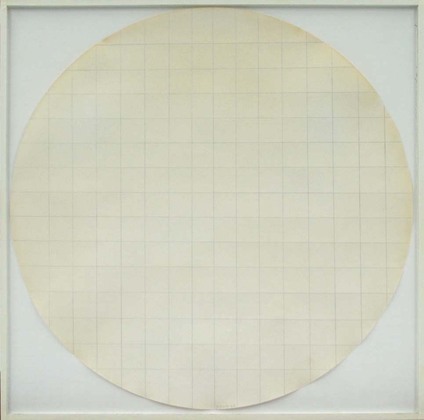The image features a minimalist piece of modern art comprising a light turquoise, slightly bluish square tile that serves as a border. At the center of this square tile, there is a prominent circular element, resembling a paper cut-out. This circle, with a subtle yellowish off-white or cream hue, has a grid pattern of light grayish-blue lines that meticulously extend across its surface. Each line within the circle forms a series of small, perfectly measured squares or rectangles. The light gray grid lines blend harmoniously with the background, yet remain distinguishable on the creamy surface. The circle touches the edges of the square frame, which appears to have a raised and beveled perimeter, adding to the textured appearance. The overall composition exudes a highly minimalist aesthetic, characterized by its simple geometric shapes and subdued color palette.